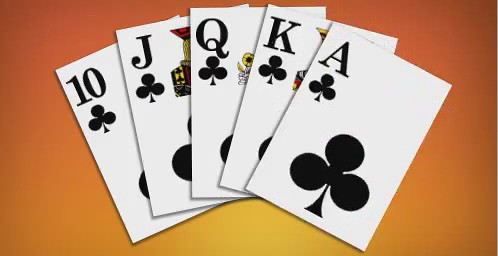This is an illustration featuring five playing cards from the Clubs suit, meticulously arranged in ascending order from left to right. The cards overlap partially, forming an elegant arc reminiscent of how they might appear if held in a player's hand. The sequence starts with the Ten of Clubs, followed by the Jack of Clubs, the Queen of Clubs, the King of Clubs, and finally, the Ace of Clubs. Each card is depicted with crisp, clear details, and is set against a vibrant orange background that adds a striking contrast to the dark, distinct motifs of the black clubs. The overall appearance suggests a digitally generated image rather than a traditional photograph, capturing the essence of a perfect hand in a stylized and visually engaging manner.